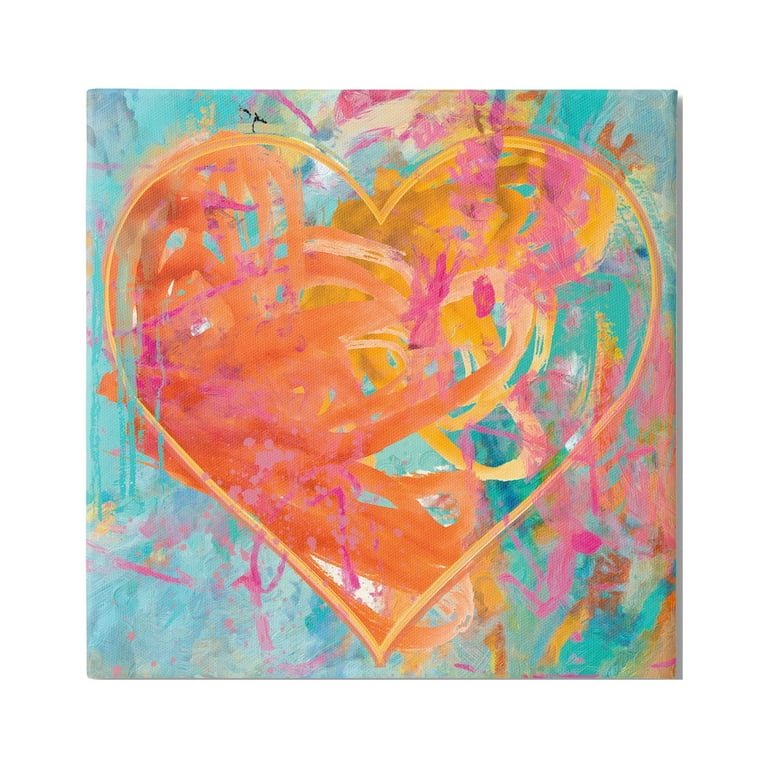This artwork showcases a predominantly abstract painting on a square canvas, where the main feature is a perfectly outlined, hollow heart. The heart, distinct and done primarily in light orange with red and white accents, stands out against a vibrant background. The backdrop is a blend of smears and splashes of baby blue, dark blue, pink, orange, gold, red, brown, and green, creating a dynamic and textured composition that looks like it was finger-painted. Within the heart and around it, the colors blend into each other with exuberant swashes, dominated by shades of light red, orangish-yellow, and pink, with occasional splashes of black, white, and a notable blue dot. The entire aesthetic is abstract except for the clear and precise heart shape in the center.